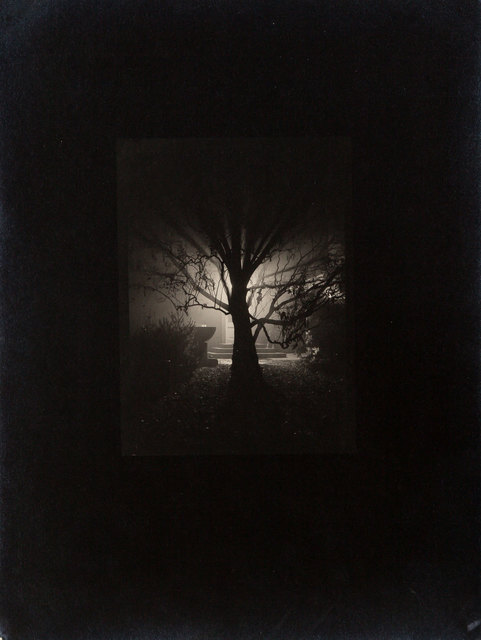A haunting, black-and-white photograph evokes a vintage film noir aesthetic. It features an elongated vertical frame dominated by a pitch-black background, within which a small, off-tone brownish rectangle reveals the actual scene. At its center stands the silhouette of a barren, scraggly tree, devoid of leaves, outlined only by the faint backlighting from an indistinguishable light source, possibly a porch light, positioned behind it. The light barely illuminates three rounded steps leading up to what could be the front door of a house, shrouded in darkness. To the left of the tree, there's a structure resembling a bird feeder or planter, hinting at an eerie, abandoned ambiance. Further details emerge, such as faint outlines of bushes in the corners and scattered leaves on the ground, completing the picture's nocturnal, desolate feel.